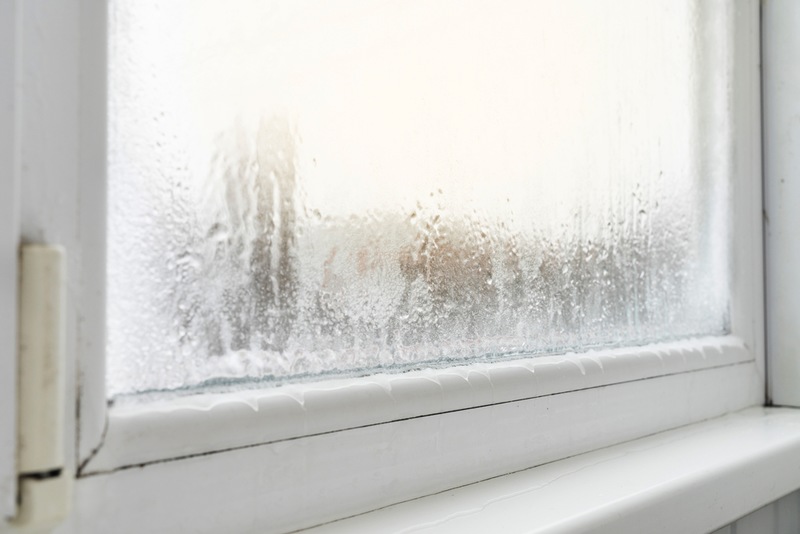This photograph captures a frosty, ice-covered window taken from the outside of a house. The windowpane is heavily blurred by the frost and condensation, making it impossible to see through to the other side. Icicles and droplets of frozen water have formed at the base of the window, suggesting the pane is not fully sealed. The window is framed by a white windowsill, which extends outward and is surrounded by a white frame. To the lower right, a triangle of light grey, painted wood siding—presumably part of the house—can be seen. The wintry scene outside includes falling snow and a blanket of ice enveloping the surroundings, creating a stark and chilly atmosphere.